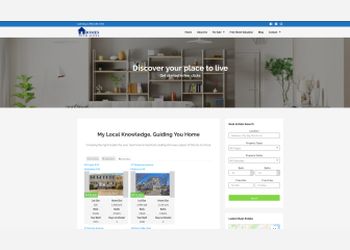A screenshot of a website with a pixelated resolution, revealing a predominantly white color scheme accentuated by blue and green elements. At the top left, there is a blue house logo accompanied by unreadable text. The navigation bar contains six tabs for site navigation. Above it, a slim blue bar likely contains social media links.

The banner image is a rectangular photograph depicting a neatly arranged interior shelf adorned with plants. Overlaying the image is the readable slogan: "Discover your place to live." Below, there is additional blurred text followed by a phrase partially legible as "My local knowledge, guiding you...".

Further down, there are images of two buildings, each accompanied by unreadable descriptive text. To their right, there is a form comprising seven fields, possibly for filtering options or sign-up purposes, topped with an unreadable large green button. The bottom part of the screenshot hints at an embedded maps widget, though it is cut off and not fully visible.